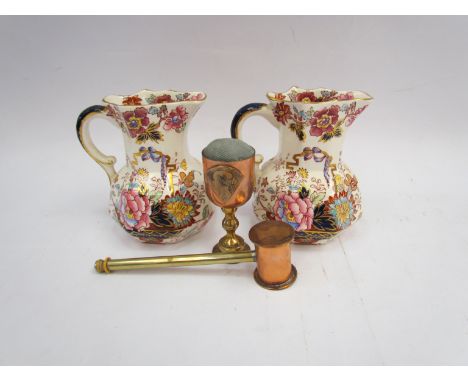The image depicts an off-white background showcasing two identical ceramic vases adorned with intricate floral patterns. These vases, resembling pitchers or jugs, are placed side by side on a white surface. Between them stands a small, golden chalice containing an indeterminate gray substance, possibly plastic. In front of the chalice lies a gold-colored mallet, reminiscent of a gavel used in courtrooms. The overall scene appears antique, accentuated by the detailed decorations on the vases, which include small points and ribbons.